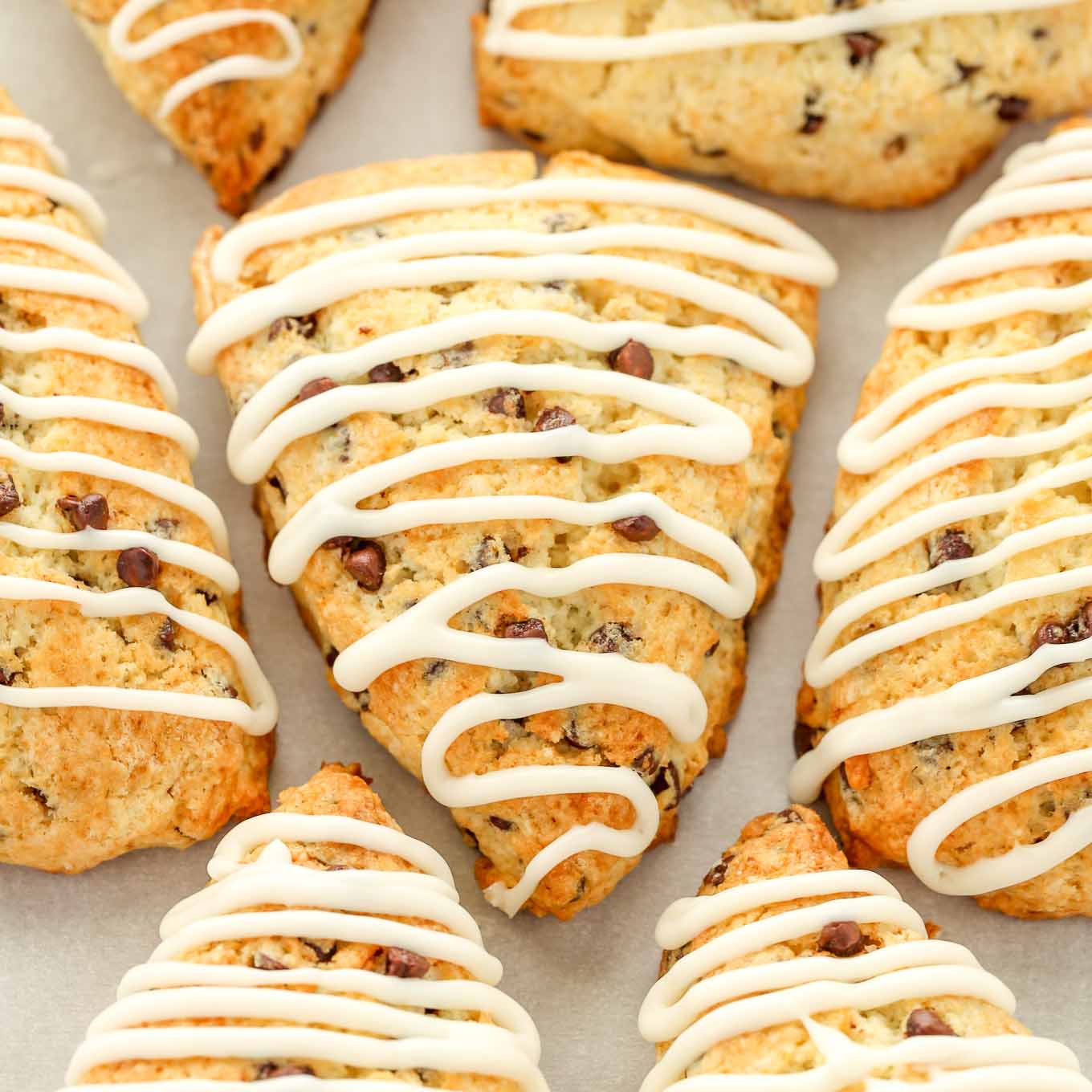The close-up, color photograph presents a tantalizing display of freshly baked chocolate chip scones, drizzled with white icing in a zigzag pattern. Set against a bright and naturally lit background, the triangular scones, golden brown with visible chocolate chips, suggest a perfectly baked texture — soft yet slightly crisp. The image, in portrait orientation, showcases a total of five scones, with the central scone fully visible. The surrounding scones are partially cropped at the edges, enhancing the intimate, close-up perspective. The scones rest on a white tabletop, with the possible subtle presence of sheet paper beneath them, adding to the realism and home-baked charm of the scene. The photograph, capturing the deliciously detailed features of the scones, exudes a sense of readiness to be enjoyed.